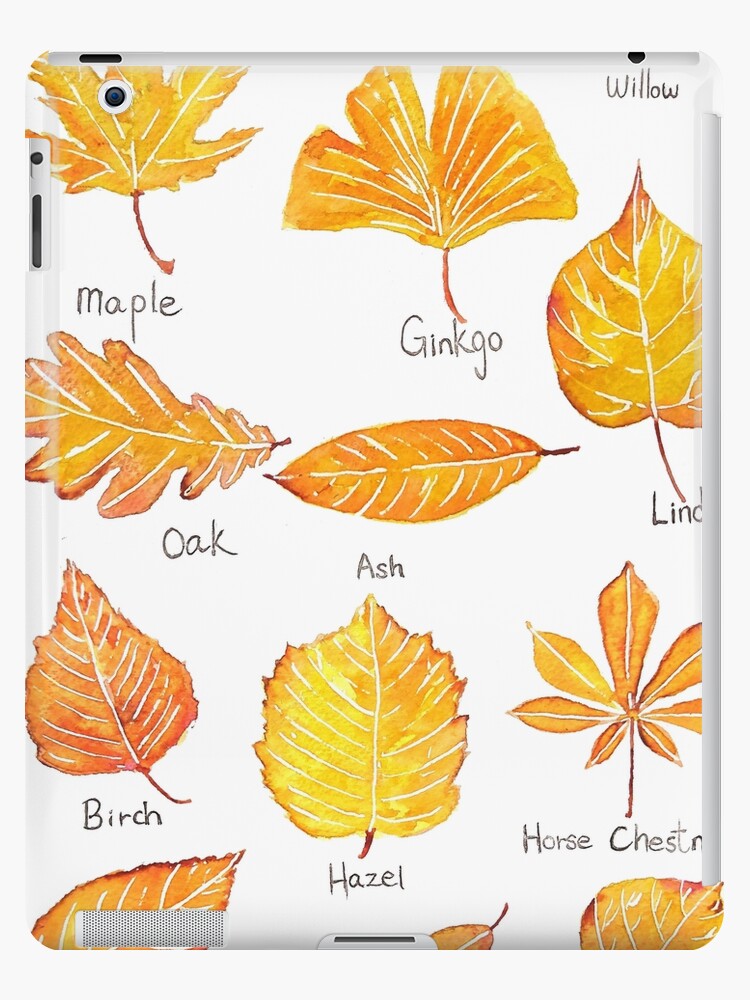This color photograph depicts a white iPad or tablet cover adorned with various hand-drawn leaves, each meticulously labeled in handwritten text. The leaves, rendered in shades of yellow, orange, red, gold, tan, and black, span across the cover against the white background. At the top left, a detailed maple leaf rests above its label. Nearby, a ginkgo leaf is similarly illustrated and labeled. The cover also features leaves such as willow (partially cut off in the image), oak, ash, birch (noted for its orange hue), hazel (in yellow), horse chestnut, and several others where portions are obscured or cut off. The craftsmanship suggests a blend of both professional and amateur qualities, neither fully hyper-realistic nor overly simplistic. Practical features like a hole for the camera lens and speaker openings are evident in the upper left and lower left corners, respectively, seamlessly integrated into this artistic piece.